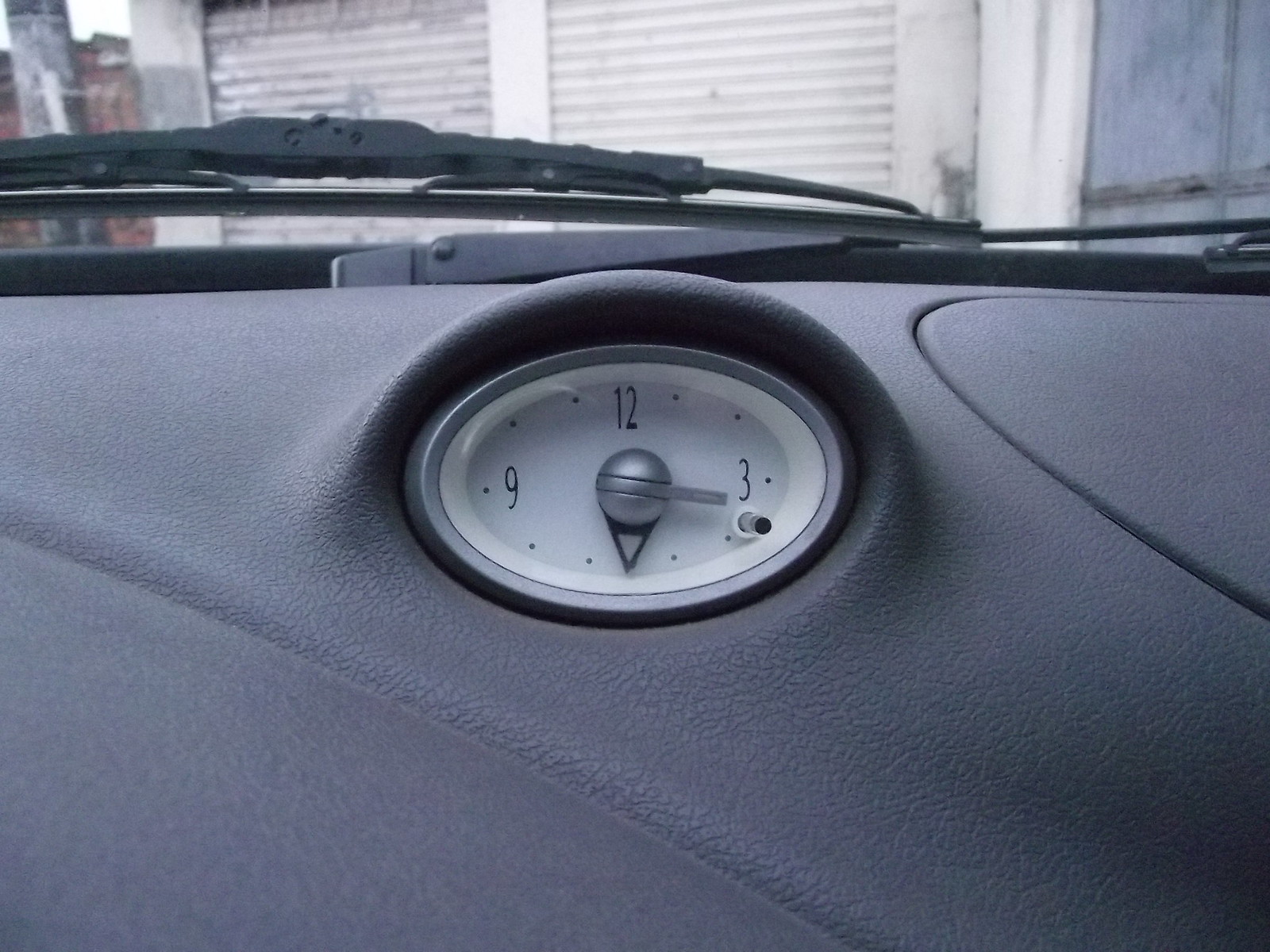This photograph captures a partial view of a car’s dashboard, focusing primarily on its upper section. The dashboard is a dark gray color, providing a contrasting backdrop for the elements on it. The central feature is a clock, which stands out with a distinctive black push button and an oval-shaped silver frame. The clock face is white, displaying the numbers 9, 12, and 3 in black, along with smaller black dots indicating the other hours.

In the periphery, parts of the windshield wipers are visible, matching the dark gray tone of the dashboard. Beyond the windshield, the view features a weathered, white, and somewhat dirty portion of a building, which includes a visible garage door. Further in the background, a brick building can be seen, completing the urban setting of this scene.